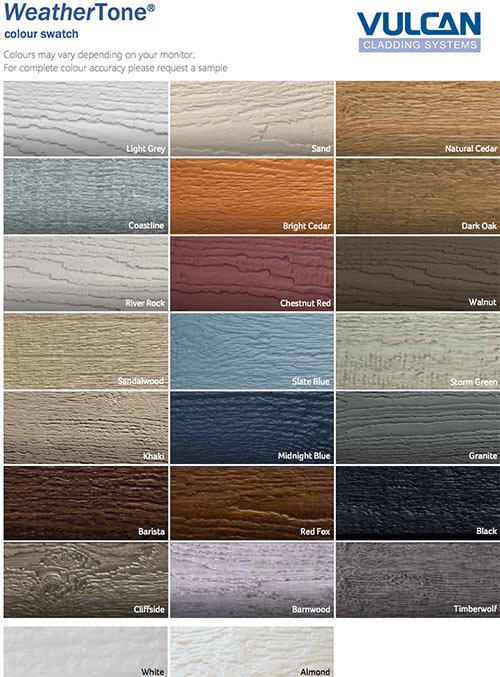This image showcases a detailed display of 24 cladding system color swatches arranged in a grid of three columns and eight rows. Titled "Weather Tone Color Swatch" in blue text, the swatches range in a spectrum of colors including light gray, sand, natural color, coastline, bright cedar, dark oak, river rock, chestnut red, walnut, sandalwood, slate blue, storm green, khaki, midnight blue, granite, barista, rice fox, black, cliffside, barnwood, thimble, white, and almond. Each swatch features a textured appearance, simulating the look of wood. The right side of the image is branded with "Vulcan Cladding Systems." A note below advises that colors may appear differently on different monitors and recommends requesting a sample for accurate color matching. Each color name closely reflects its actual hue, providing an accurate visual guide for potential buyers.